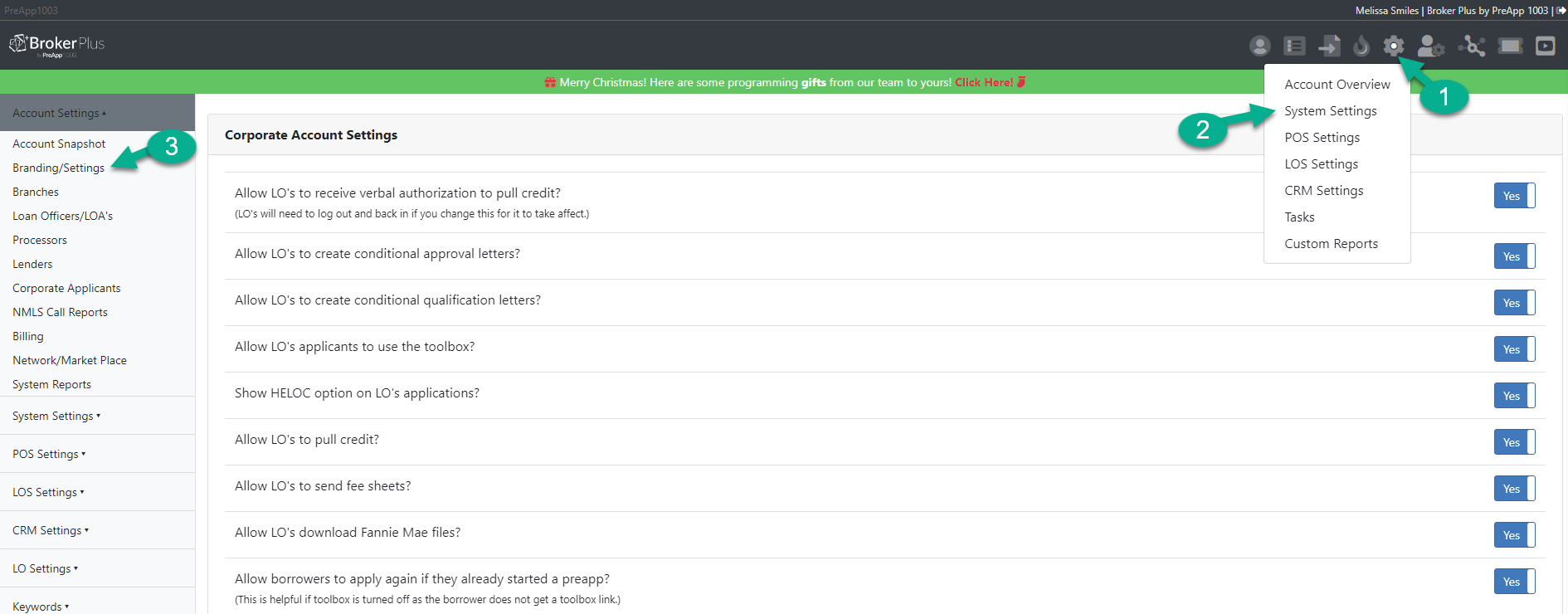The screenshot depicts a software interface for a platform named "Broker Plus." On the left-hand side, a sidebar lists several account settings options. The image contains multiple labeled arrows guiding the user through the interface: 

1. A red arrow labeled "1" points to the general account settings section.
2. A blue arrow labeled "2" directs attention to the system settings.
3. A green arrow labeled "3" highlights the branding settings.

Additionally, there is a section labeled "Corporate Account Settings" that enumerates a list of nine specific settings. Each of these settings is marked with a blue box indicating "Yes," signifying that they are all enabled. The context suggests these settings relate to permissions or configurations required for corporate branding approvals within the account setup.